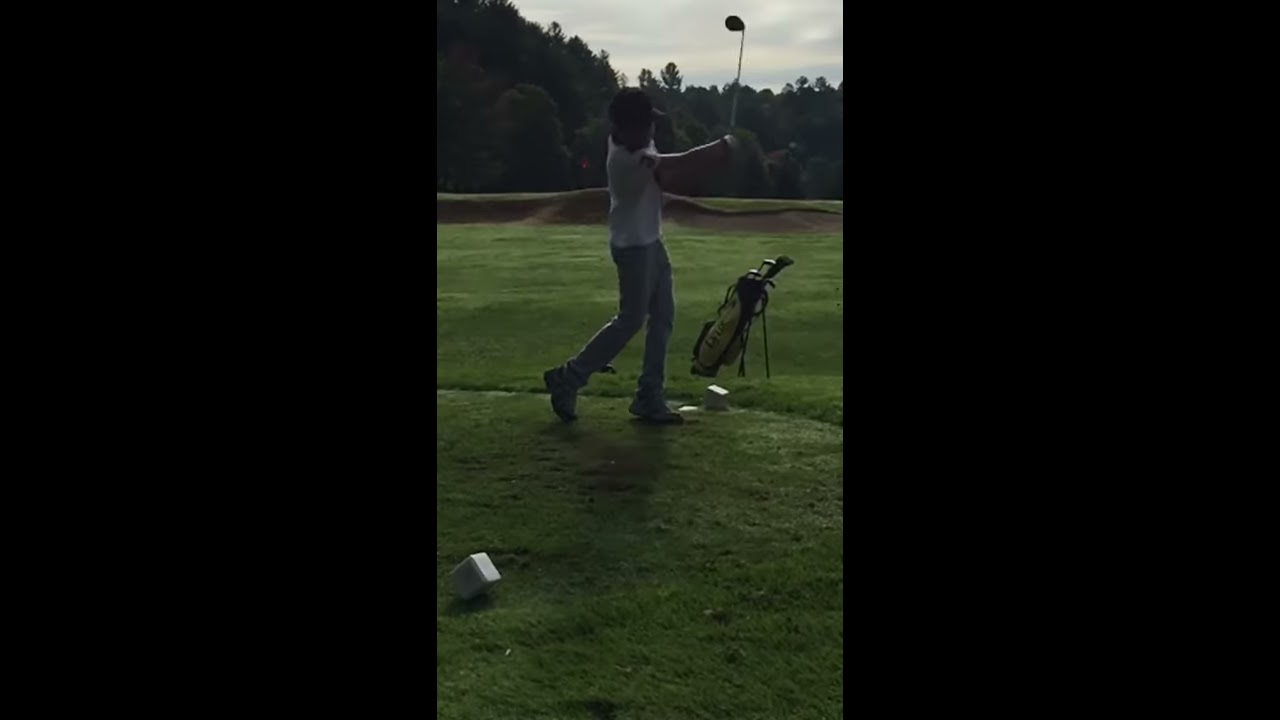The photographic triptych captures a moment on a golf course, where the central panel focuses sharply on a man finishing his golf swing. Flanked by solid black left and right panels, the vivid center image stands out. The man, wearing a cap, gray shirt, and dark pants, is positioned on a lush green, facing right. His golf club is raised high, perpendicular to the ground, indicating the completion of a strong swing. His golf bag, balanced on a tri-stand, is visible behind him with club heads peeking out. The background features a lush, wooded area filled with dense trees, and the sky above is bright blue adorned with fluffy white clouds. The foreground and middle ground present a carpet of grass, while beyond the man, sand bunkers highlight the golf course's landscape. The overall composition is a balanced blend of detailed action and serene surroundings.